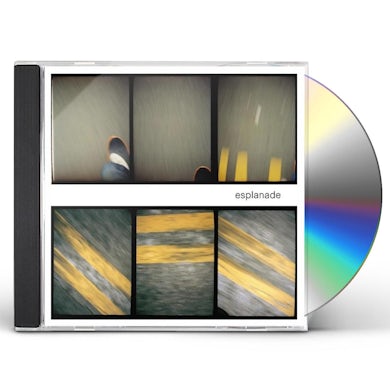The image displays a CD jewel case against a white background, with approximately one-third of the CD disk emerging from the right side of the case. The black spine on the left contrasts with the detailed cover art on the front. The artwork is divided into six quadrants. The upper three quadrants resemble a film strip, featuring a person's feet on a brownish road with yellow double lines. The lower three quadrants focus on close-up views of yellow road markings on a dark background. Between the upper and lower sections, there's a white gap containing the text "Esplande."